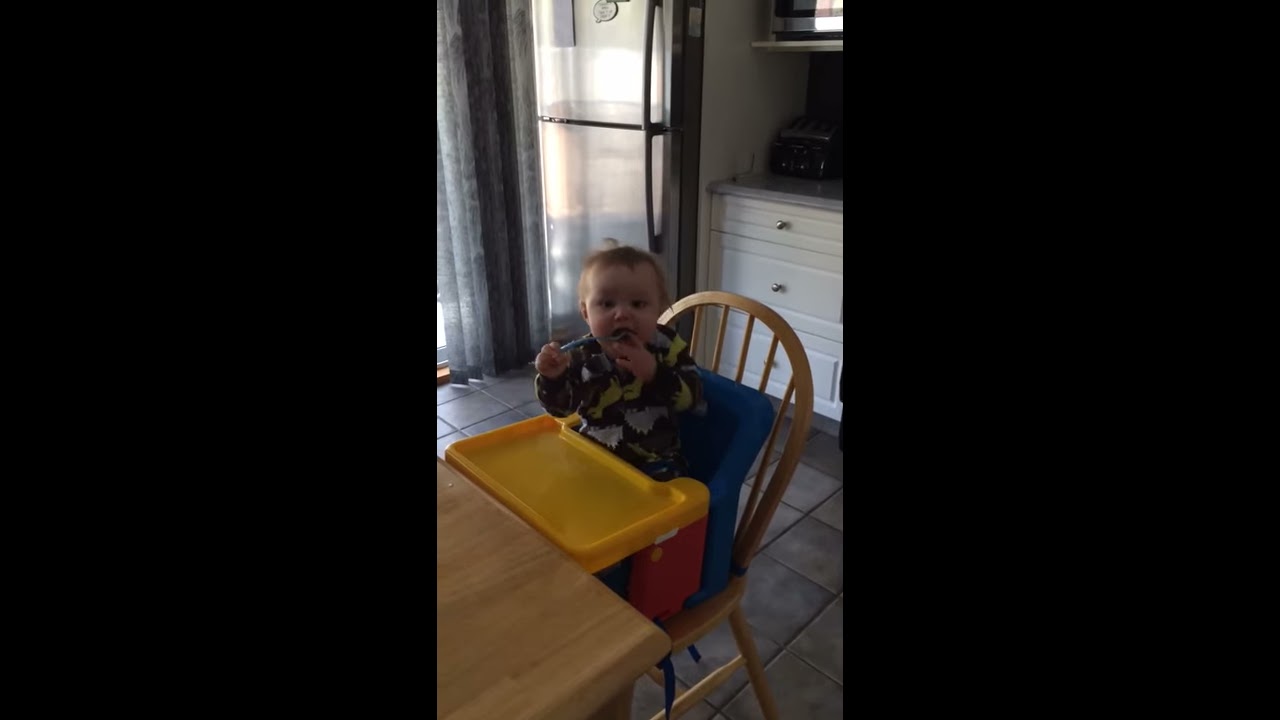The image shows a baby, likely under a year old, seated in a blue and red plastic high chair with a yellow tray, which is placed on a light wooden kitchen chair with spindle back design. The baby is positioned at a matching wooden table in the center of a kitchen with gray tile flooring. He is wearing a blue sweater adorned with yellow and multicolored fish, and he is holding a spoon. The kitchen in the background features white cabinets with three visible drawers, a stainless steel refrigerator with a top freezer, and a countertop with a toaster. To the left of the refrigerator, there is a window with curtains, possibly covering a sliding glass door. The scene is brightly lit, suggesting it is daytime, and the overall setting suggests the baby is ready to be fed.